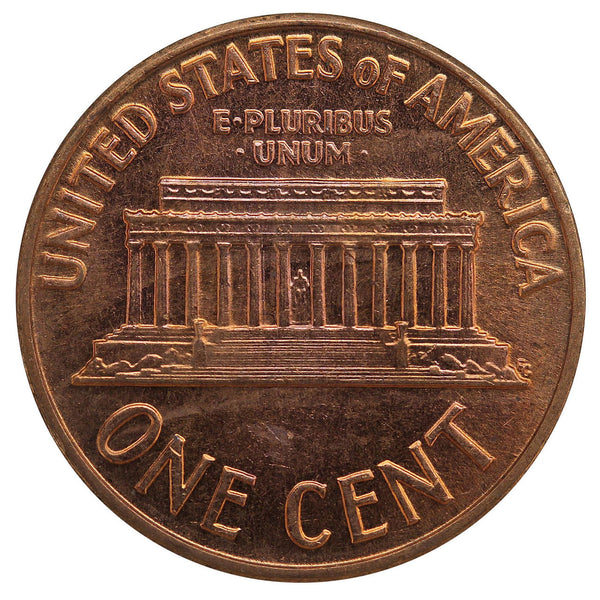This close-up image is of the reverse side of an American penny, amplified without any definitive background, much like an enlarged product view seen online. The copper-colored coin features the text "United States of America" curved along the top edge. Directly beneath it, the Latin phrase "E Pluribus Unum" is inscribed. Centrally displayed is the Lincoln Memorial, characterized by its recognizable columns, steps, and the seated sculpture of Abraham Lincoln visible inside the monument. At the bottom edge, the text "One Cent" is also curved along the rim of the coin. The penny displays minor signs of wear with slight fading and scratching but remains identifiable by its smooth rim and classic design. The photograph isolates the coin, emphasizing its familiar details and texture.